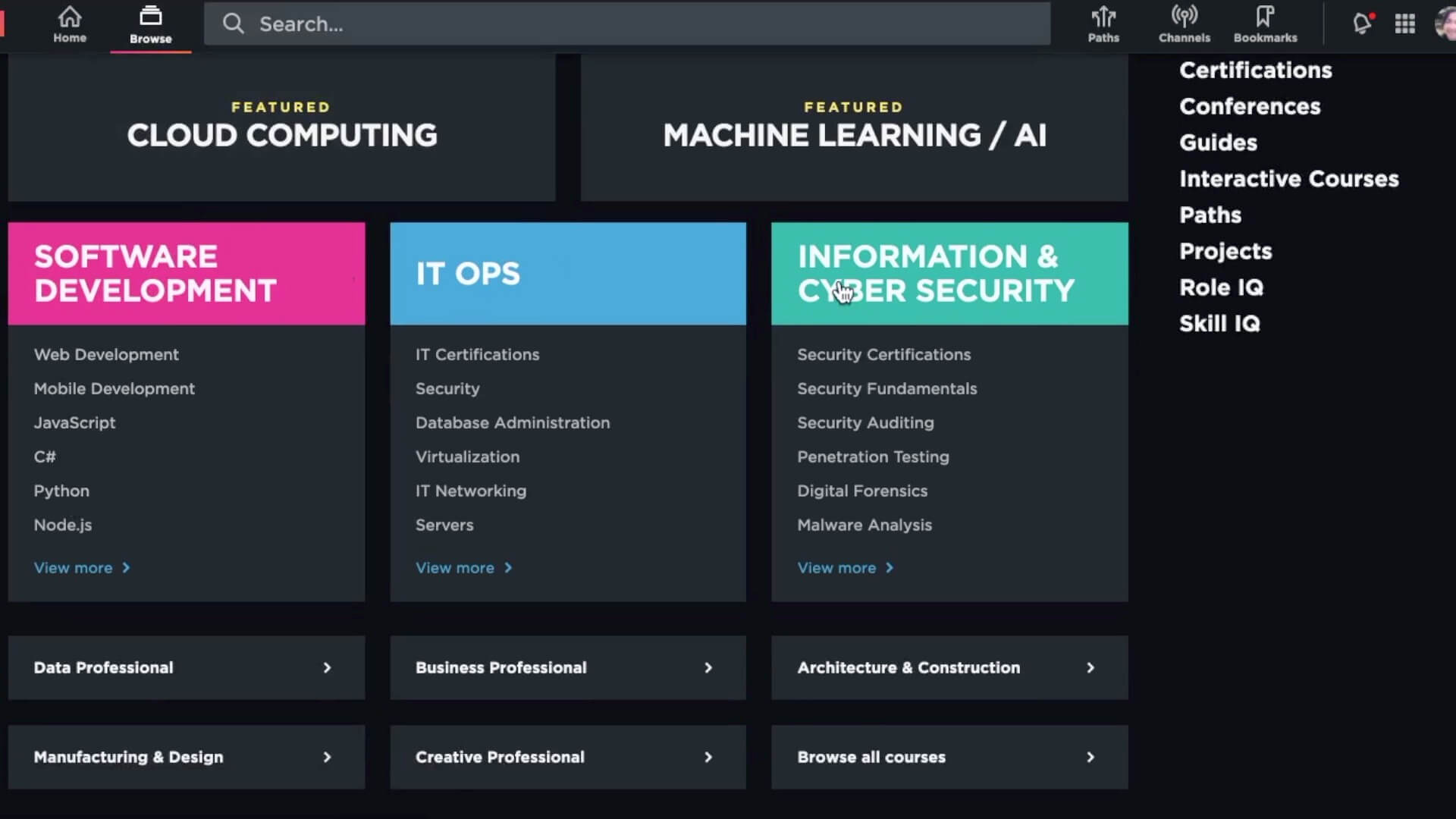This image captures a website interface featuring a predominantly black and gray color scheme. In the upper left corner, within a black bordered section measuring approximately half an inch tall and extending two inches from left to right, there is a home icon labeled "Home," directly beneath which is a browse icon labeled "Browse." The word "Browse" appears in gray, accentuated by a red line underneath.

To the right lies a prominent search bar spanning about two-thirds of the interface's width, characterized by a dark gray inner hue. It contains the placeholder text "Search..." in light gray, accompanied by a search icon on the left side of the bar. 

On the far right corner, there's a profile picture of a girl with black hair adjacent to a grid icon consisting of four rows of three dots arranged vertically and horizontally to form a square. Next to this are several icons: a notification bell with a red dot indicator, a bookmarks icon labeled "Bookmarks," a channels icon labeled "Channels," and a paths icon labeled "Paths."

Under this upper section, on the left, reside two horizontally-aligned rectangles. The first rectangle features a small yellow text "FEATURED" above a bold, capitalized white text "CLOUD COMPUTING." The adjacent rectangle, similarly labeled "FEATURED" in yellow, presents bold white text "MACHINE LEARNING / AI."

On the right side, extending vertically down a black background, is white text listing several categories: "CERTIFICATIONS," "CONFERENCES," "GUIDES," "INTERACTIVE COURSES," "PATHS," "PROJECTS," "ROLE IQ," and "SKILL IQ." The section beneath this text remains entirely black.

Returning to the left side, three horizontally-aligned rectangles are visible. The first rectangle features a pink border and contains white text reading "SOFTWARE DEVELOPMENT," followed by additional information, separated by small spaces and tabs. The middle rectangle, set against a blue background, displays the text "IT OPS" with corresponding information structured similarly. The final rectangle, in a teal green hue, is labeled "INFORMATION AND CYBER SECURITY," also followed by pertinent details and spaced elements.